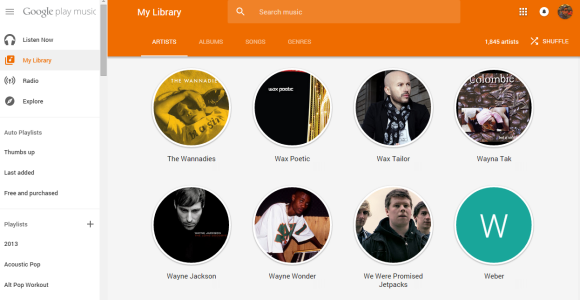The rectangular image, oriented with its long side stretching horizontally, is divided into two sections. The left-hand side, occupying roughly a quarter of the entire image, features a vertical menu column. At the very top left corner of this column is a hamburger icon, and adjacent to it is the text "Google Play Music". Below this, listed in descending order, are menu options: "Listen Now" with a headphone icon, "My Library" with a two-page icon (highlighted in orange), "Radio" with a speaker sound icon, and "Explore" (icon not clearly visible). Further down, additional menu items include "Auto-Playlist", "Thumbs Up", "Last Added", "Free and Purchased", followed by playlist names such as "2013", "Acoustic Pop", "All Pop", and "Workout".

The main body of the image to the right is topped with an orange banner. Written in white text on this banner is "My Library", accompanied by a search box and search icon. The current selection highlighted under this section is "Artists".